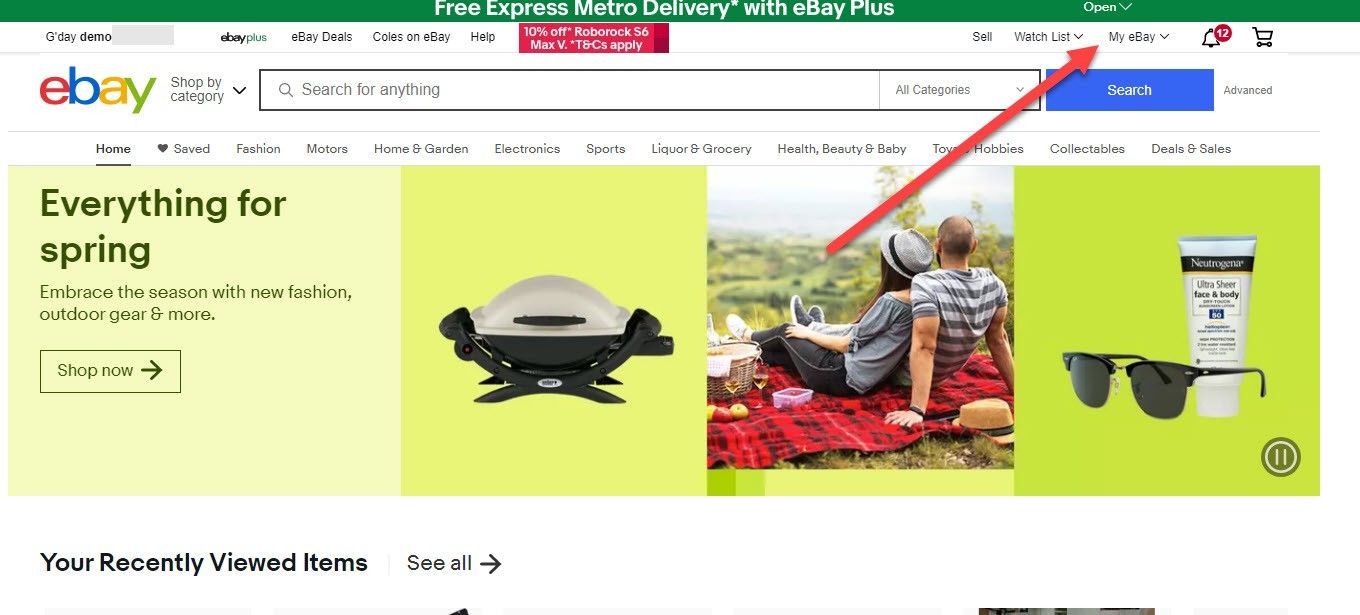This horizontally-oriented image captures a screenshot from an eBay web page, viewable on both smartphones and computers. At the top of the image, a thin green rectangular line features the text "FREE EXPRESS METRO DELIVERY WITH EBAY PLUS" in white, with smaller white font next to it stating "open" and a right-pointing arrow.

To the left, the text "G'DAY DEMO" is displayed alongside a gray, empty box. Below this, there are several navigation tabs: "eBay Plus, eBay Deals, Coles on eBay, and Help." Beneath these tabs, a red box announces "10% off" a specific item. Continuing to the right, additional navigation options include "Sell," "Watch List," "My eBay," with a reddish-orange arrow pointing to "My eBay." Nearby icons include a bell for notifications and a shopping cart.

The iconic eBay logo, with its red "e," blue "b," yellow "a," and green "y," is prominently displayed. Below the logo, there's a functional search bar allowing users to shop by category, search across all categories, and access an "Advanced" search option.

The left-side navigation provides access to various sections: "Home," which is underlined, "Saved," "Fashion," "Motors," "Home & Garden," "Electronics," "Sports," "Liquor & Grocery," "Health & Beauty," "Baby," "Toys & Hobbies," "Collectibles," and "Deals & Sales." 

An eye-catching banner in the middle of the page promotes "Everything for Spring," featuring images of a grill, people enjoying a picnic, sunglasses, and sunscreen. At the bottom of the image, a section labeled "Recently Viewed Items" appears, with an option to "See All" these items.